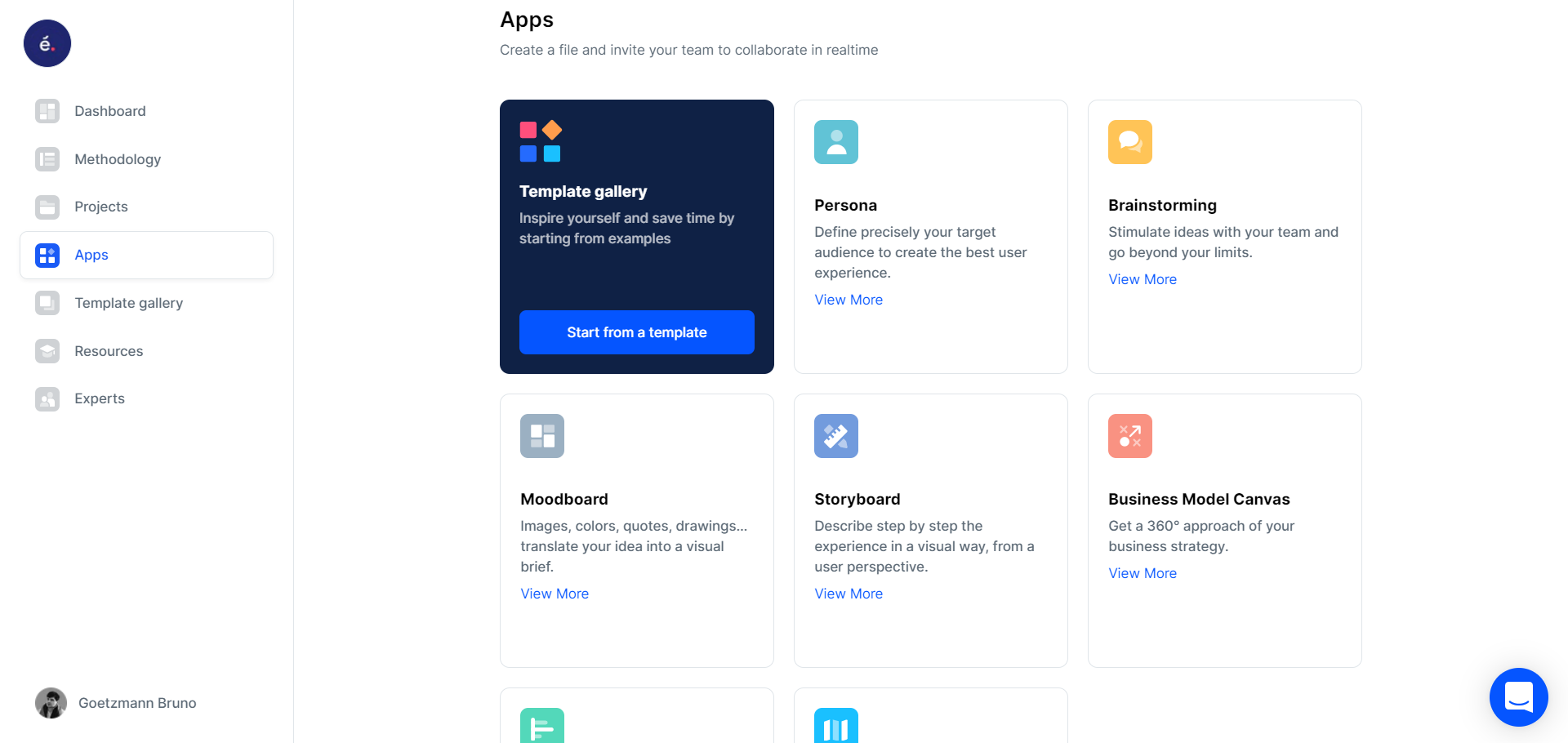The image depicts a minimalistic website named "Apps," designed for real-time collaboration and project management. The website's landing page invites users to "create a file and invite your team to collaborate in real time." The layout features a white vertical sidebar on the left, which includes navigation options like Dashboard and Market, suggesting different thematic projects possibly related to meteorology.

The "Apps" title is prominently displayed in blue along with a matching blue icon. Below this title, in the center of the main page, there is a section labeled "Template Gallery and Experts," suggesting resources for users. The Template Gallery is highlighted with a blue background, offering a starting point for users to create from predefined templates.

Adjacent to this, the page features a series of white boxes, each representing different types of project templates: Persona, Brainstorming, Mood Board, Storyboard, Business Model, Courses, and Canvas. Each template box contains a small image in its upper left-hand corner, varying in colors such as blue, green, gray, orange, and teal, providing visual cues. Users can click on these templates to initiate various projects, facilitated by the app's collaborative features.